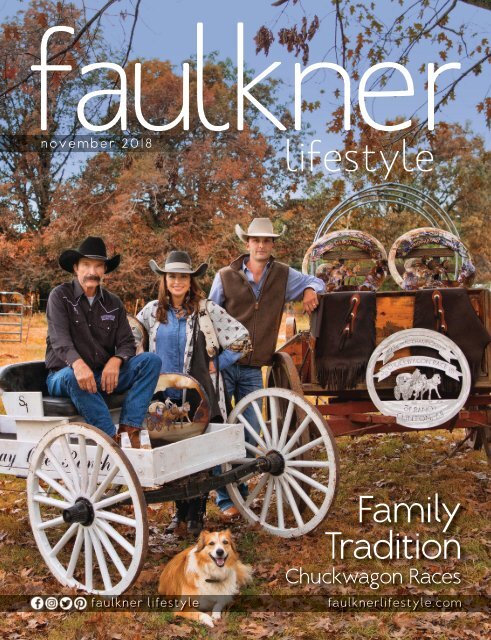The cover of the November 2018 issue of Faulkner Lifestyle magazine showcases a picturesque autumn scene with three individuals and two wagons. The featured characters are all wearing cowboy-style hats. An older man, dressed in a black long-sleeve shirt, jeans, boots, and a black cowboy hat, sits in a smaller white wagon with large white wheels. Next to him stand a woman and a younger man. The woman, sporting a gray hat with a white band, wears a blue shirt under a gray and white coat. She has brown hair. The younger man, leaning against a larger brown wagon, is clad in a blue denim shirt, a brown vest, and blue jeans, and he wears a whitish-tan cowboy hat. Adding to the charm of the scene is an orange and white collie dog sitting in front of the white wagon. The ground is scattered with fall leaves, and the trees behind them display vibrant autumn colors. The cover headline promotes a feature on "Family Tradition, Chuck Wagon Races," encapsulating the essence of the periodical's focus on lifestyle and tradition.